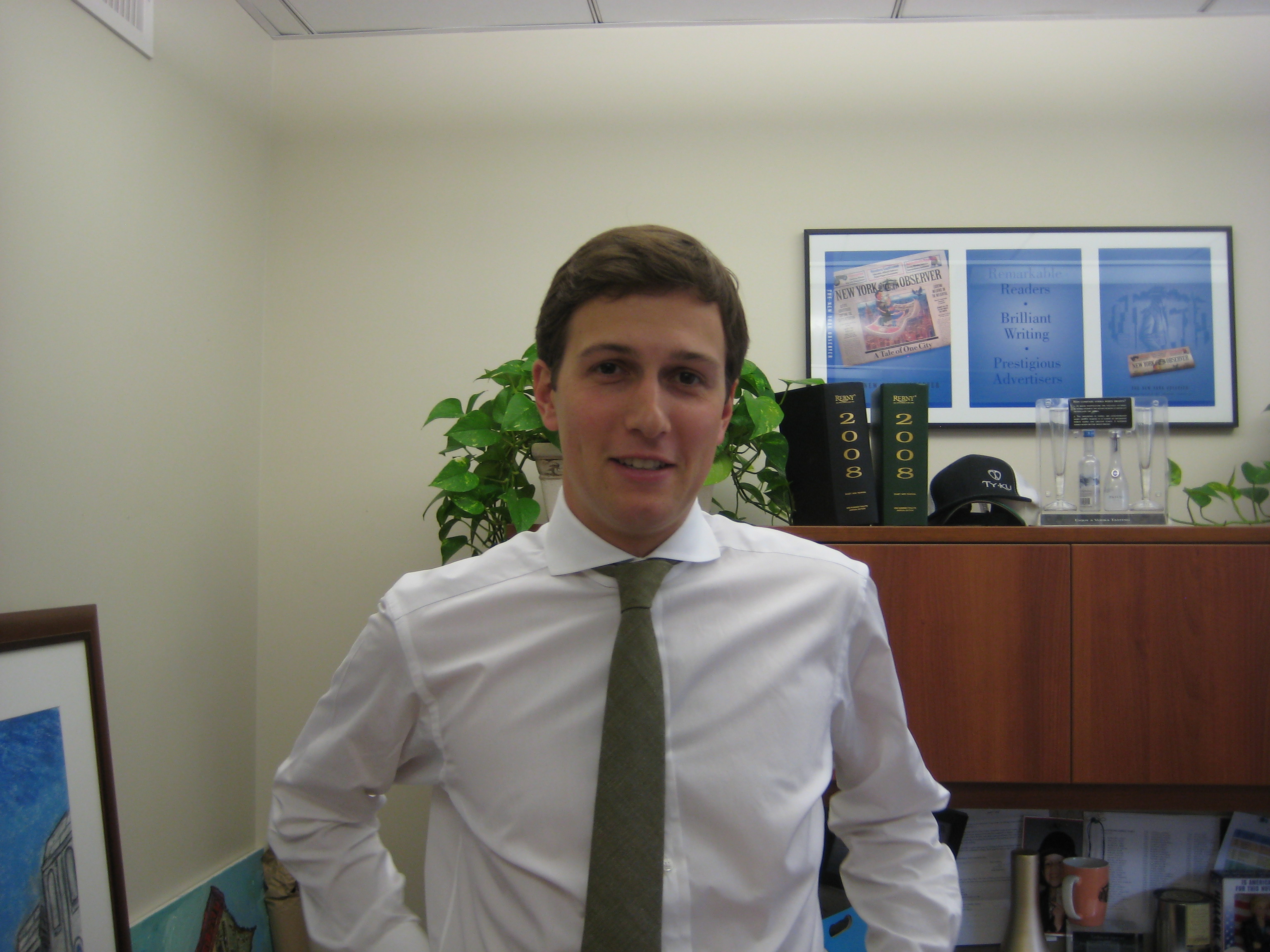In this detailed image, a young man, identified as Jared Kushner, is standing in an indoor setting that appears to be an office. He is dressed in a white dress shirt paired with a dark green necktie and is seen staring straight ahead into the camera with a slight smile. He has short, dark brown hair and brown eyes. 

Behind Jared, there is a distinctive brown shelf that houses several items, enriching the background details. Prominently, there are two large green books with gold text reading "Theory 2008" on their spines. An office plant with green leaves is visible behind his head. Next to the books, there is a baseball cap and a case containing what looks to be bottles of alcohol and a couple of wine glasses with a note on top. Below the shelf, objects such as coffee cups, papers, and photos are scattered around, adding to the cluttered yet active office environment. Additionally, a couple of paintings are seen propped against the wall to his left.

The wall in the background is white, and there is a framed photograph of a newspaper along with several other photos hanging on it, on his right. The upper side of the image reveals a portion of the ceiling and a vent located at the top left corner, completing the indoor scene's detailed depiction.